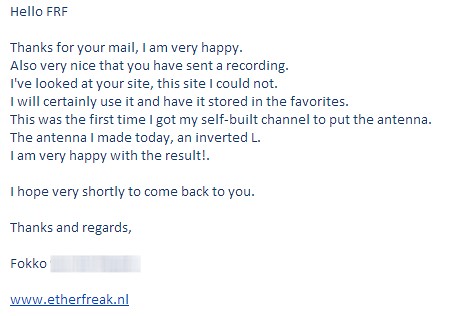The image is a screenshot of an email with black text on a white background. The email opens with "Hello FRF," followed by a message of gratitude: "Thanks for your mail. I'm very happy." It continues with appreciation for a recording received: "Also very nice that you have sent a recording." The sender mentions their attempt to explore a website: "I've looked at your site. This site I could not." They express intentions to use the site: "I will certainly use it and have it stored in the favorites."

The sender then describes their recent experience: "This was the first time I got myself a built channel to put the antenna. The antenna I made today, an inverted L. I am very happy with the result!" They express a desire to maintain communication: "I hope very shortly to come back to you."

The email concludes with "Thanks and regards," followed by the sender's name, "FOKKO," with the last name blurred out. At the bottom, there is a clickable hyperlink in blue text: "www.etherfreak.nl." The entire message is written on a plain white background.